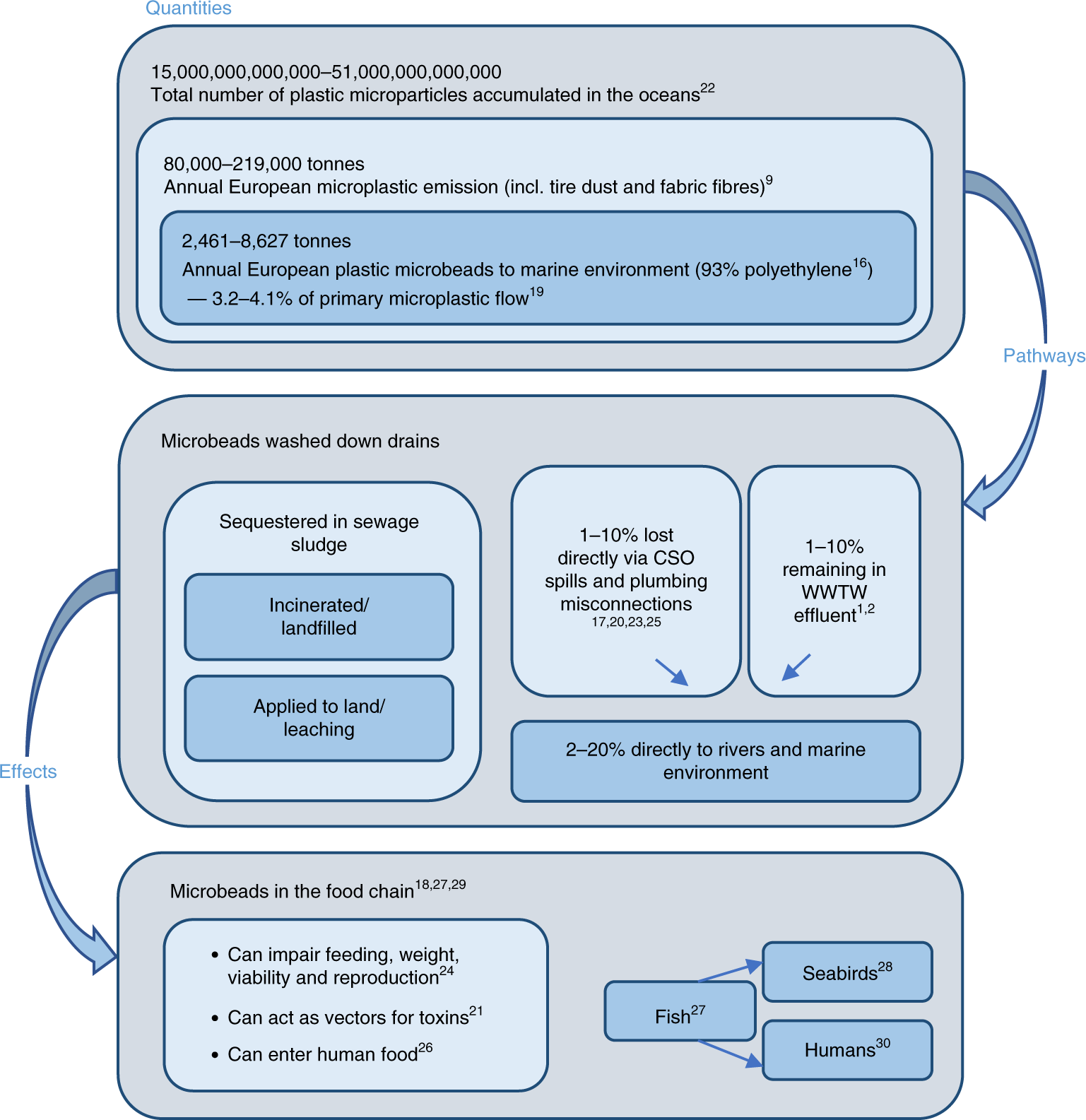This detailed image is of a comprehensive flowchart in shades of blue and gray, detailing the accumulation and impact of microplastics in the oceans. At the top, it reveals staggering quantities of plastic microparticles, with 15 trillion to 51 trillion pieces accumulating in the oceans, and between 80,000 to 219,000 tons representing annual European microplastic emissions, which include tire dust and fabric fibers. This section is followed by statistics on annual European microplastic flows to the marine environment, noting that 93% of these are polyethylene microbeads, ranging from 2,461 to 8,627 tons annually.

The flowchart traces the pathways of these microplastics, starting with microbeads washed down drains. From there, they follow paths like being sequestered in sewage sludge, incinerated or sent to landfills, or applied to land—where leaching can occur. It highlights that 1% to 10% of microplastics are lost directly via CSO spills and plumbing misconnections, with another 1% to 10% remaining in wastewater treatment works effluents, and 2% to 20% ending up directly in rivers and the marine environment.

The next segment focuses on the effects of microplastics within the food chain. It describes how microplastics impair feeding, weight, viability, and reproduction in marine life. Additionally, these particles can act as vectors for toxins and eventually enter human food. The diagram specifically points out how fish consume these microplastics, which are then ingested by seabirds and humans, highlighting the alarming interconnectedness and implications for the entire ecosystem. The image effectively uses blue arrows to illustrate these flows and impacts, reinforcing the critical message with striking quantitative data.